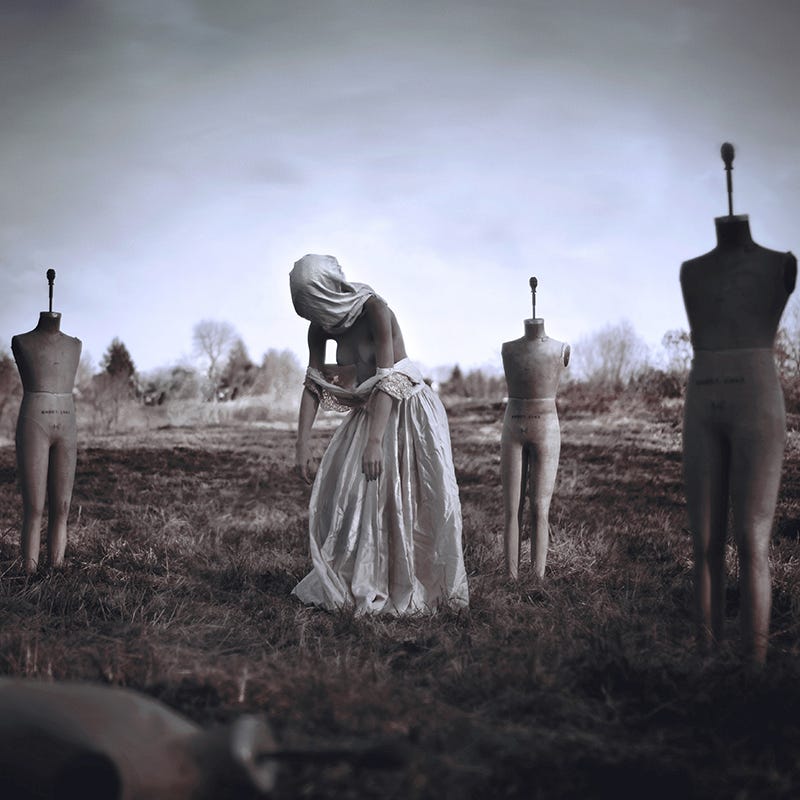In this haunting black-and-white photograph, an eerie scene unfolds in a desolate, murky field under a gray winter sky with dead, leafless plants resembling tumbleweeds. The focal point is a hunched-over woman with a white shroud covering her head and face, rendering her faceless and distressed. She stands bare-shouldered and bare-breasted, her white wedding dress slipping off her elbows, exposing her chest. Surrounding her are four headless and armless mannequins, each with a stick protruding from their necks, emphasizing the surreal and ominous atmosphere. One additional mannequin lies on the ground nearby, adding to the sense of abandonment and desolation. The entire scene is reminiscent of a post-apocalyptic tableau, capturing a harrowing, solitary moment of human fragility amidst ghostly, inanimate figures.